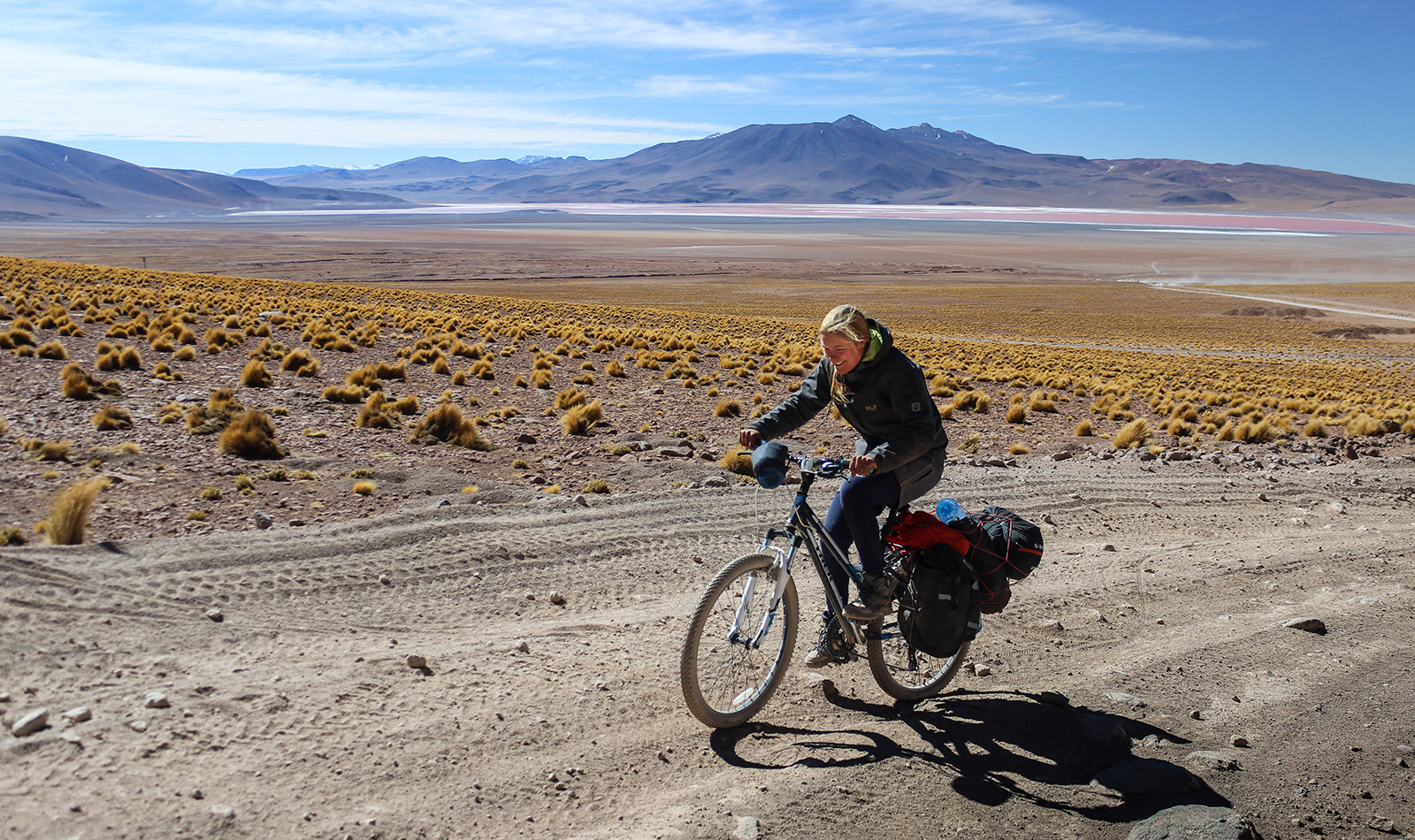In this vibrant and detailed outdoor scene, a woman, donned in a dark-colored jacket, jeans, and shoes, rides a mountain bike on a dirt road that cuts across a dry, arid landscape. Positioned slightly to the right of center in the lower section of the image, she is pedaling from right to left, her bike angled towards the viewer. Her blonde hair peeks out from under an unidentified head covering, possibly a cap, and she beams a big smile, her hands firmly gripping the handlebars as if she might be navigating a slight incline. The bike is loaded with bags attached to the rear, hinting at a journey or adventure.

The dirt road she travels winds from the bottom left of the image, subtly rising and ending midway on the right side. Surrounding her, the terrain is flat and barren, speckled with patches of yellow-brownish clumps of grass or weeds. The plain stretches out towards a distant horizon where large hills or mountains rise against a backdrop of a bright blue sky scattered with white clouds. The clarity of the image underscores the stark yet captivating beauty of this sunlit and expansive landscape.